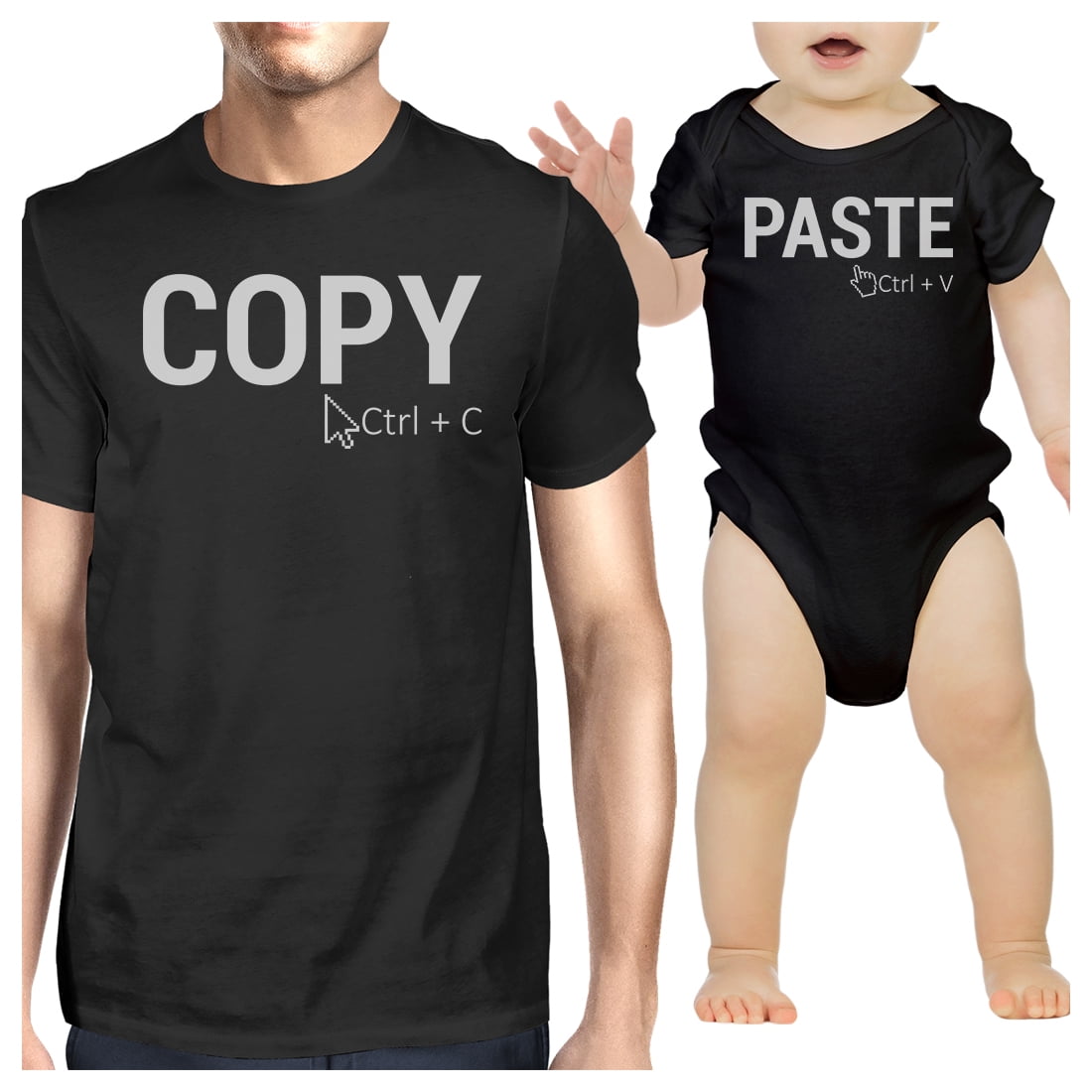The image is a commercial showcasing coordinated apparel for an adult and baby. The adult is wearing a black t-shirt featuring the phrase "Copy Ctrl+C" along with a mouse icon, while the baby, standing, is dressed in a matching black onesie with the phrase "Paste Ctrl+V." Both texts are printed in large, bold white letters, emphasizing the playful concept that the child is a "copy" of the parent. The photograph predominantly focuses on the shirts, showing the adult's back and lower chin, and both figures are against a clean, white background, highlighting the message and matching outfits.